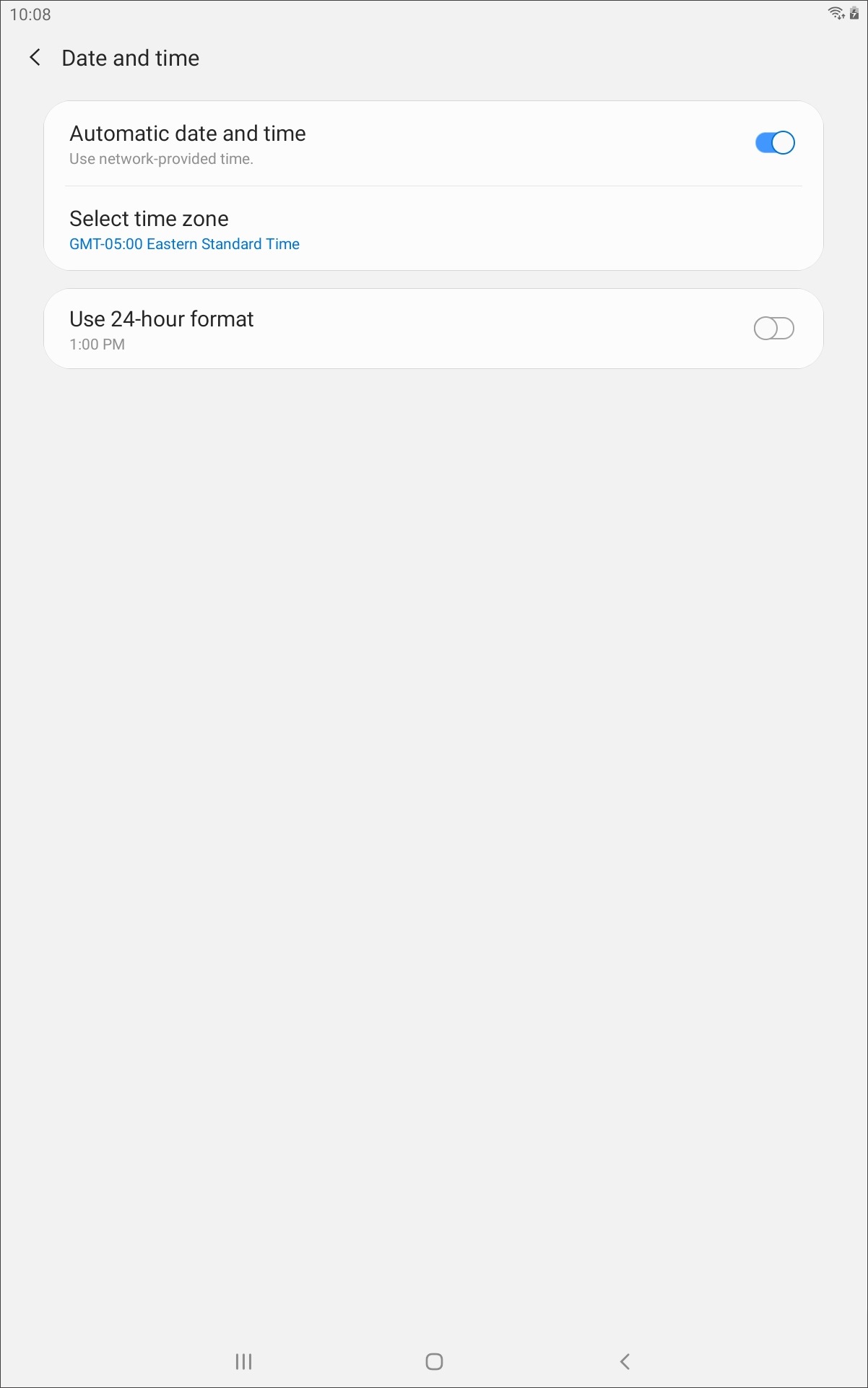The image depicts the date and time settings screen of a tablet. The screen is divided into distinct sections with a primarily light gray background. At the top left corner, the time is displayed as 10:08. On the top right corner, Wi-Fi, data signal, and a battery charging icon (showing it's half full) are visible.

The main content area starts with a section labeled "Date and time" accompanied by a left-facing arrow. Below this, the option "Automatic date and time" is listed with the description "Use network-provided time," which is toggled on, indicated by a blue switch. 

Following that, there's the "Select time zone" option displayed in black text, showing "GMT-05:00, Eastern Standard Time" in blue text. Below this is the option "Use 24-hour format," currently toggled off, and showing an example time of "1:00 PM."

The entire page is encased in a very thin black border surrounding the screen. At the bottom of the screen, three navigation icons are present: three horizontal lines, a square, and a backward-facing arrow, all colored in black. The fields for "Automatic date and time," "Select time zone," and "Use 24-hour format" have white backgrounds, standing out against the overall light gray background of the screen.

The layout is clean, with plenty of negative space for easy readability, highlighted by the contrast between white data fields and the light gray background.